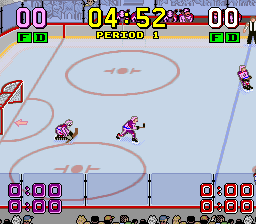The image is a pixelated screenshot of a retro-style hockey video game. On the left side of the white ice hockey rink, three players are positioned, all facing right. One player appears to be crouching with a hockey stick, while another skates ahead. In the upper right corner, a referee can be seen, with an additional skater slightly below. The red goal net, with detailed mesh, is situated on the far left of the rink. Surrounding the rink, pixelated spectators watch the game, adding to the nostalgic feel of the graphics. At the top of the screen, the score reads "00 FD" in purple for one team and "00" in white for the other team, with the current period time displayed in yellow as "04:52" for period one. The bottom corners of the screen show redundant timing or scores, depicted as "0:00" in purple on the left and red on the right, respectively.